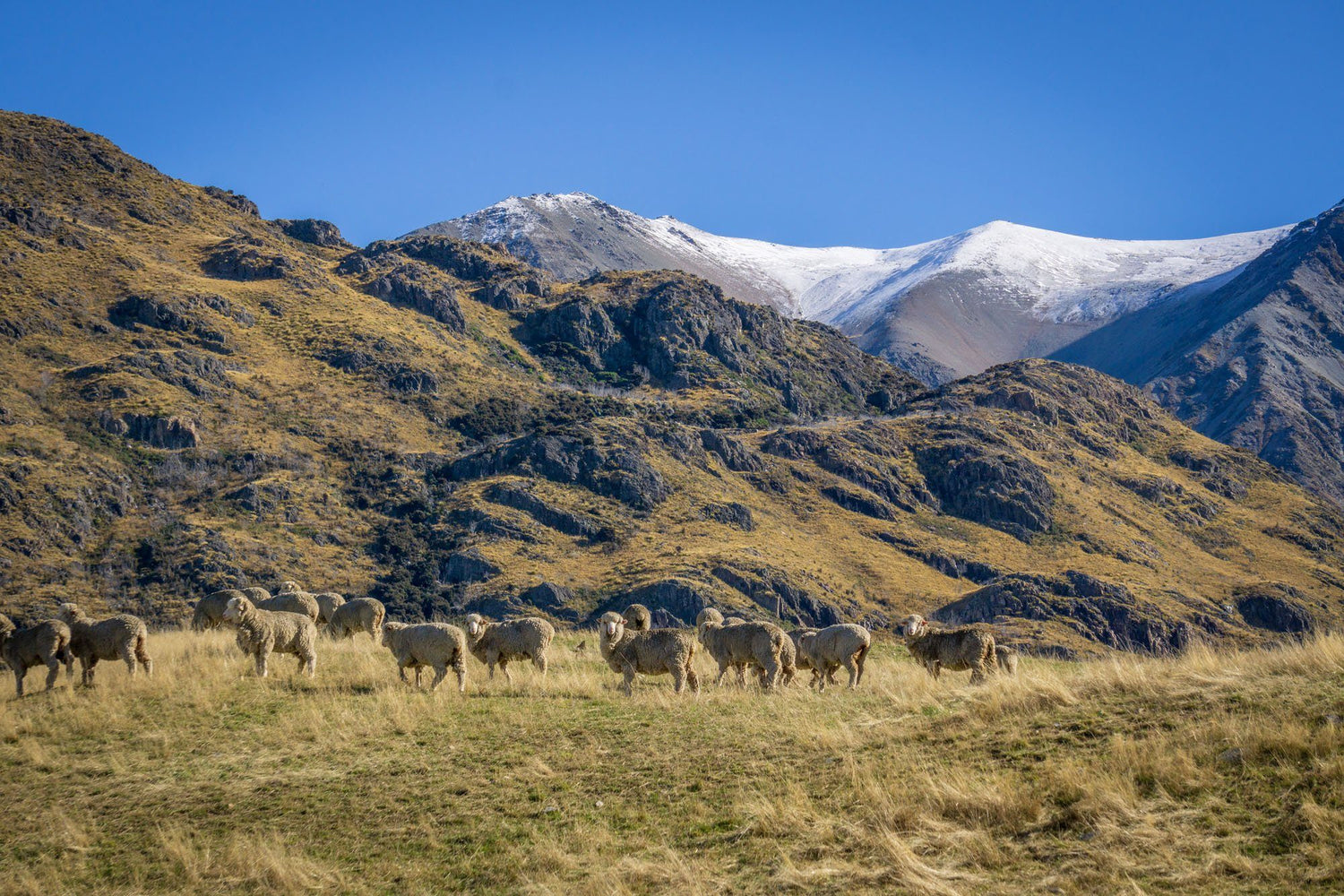In this captivating daytime photograph, a serene pastoral scene is depicted with a herd of approximately 15 tan-colored sheep scattered across a grassy field. The sheep, which all possess thick wool and predominantly face left, are positioned on varying grass heights, suggesting some areas have been grazed more than others. The verdant field shows patches of lush green interspersed with some brown areas, indicating natural wear. The image is rich with color, showcasing shades of white, gray, brown, tan, beige, and dark green. 

In the backdrop, a range of mountains rises majestically. The closest mountains exhibit a mixture of grassy and rocky textures, while a distant range features striking black rock sections capped with pristine snow, evoking a sense of cold and serene beauty. Above this picturesque landscape, the sky stretches out, enhancing the tranquil and wild nature of the scene. This photograph unmistakably captures the essence of a remote, natural area where the presence of snow suggests a colder climate.